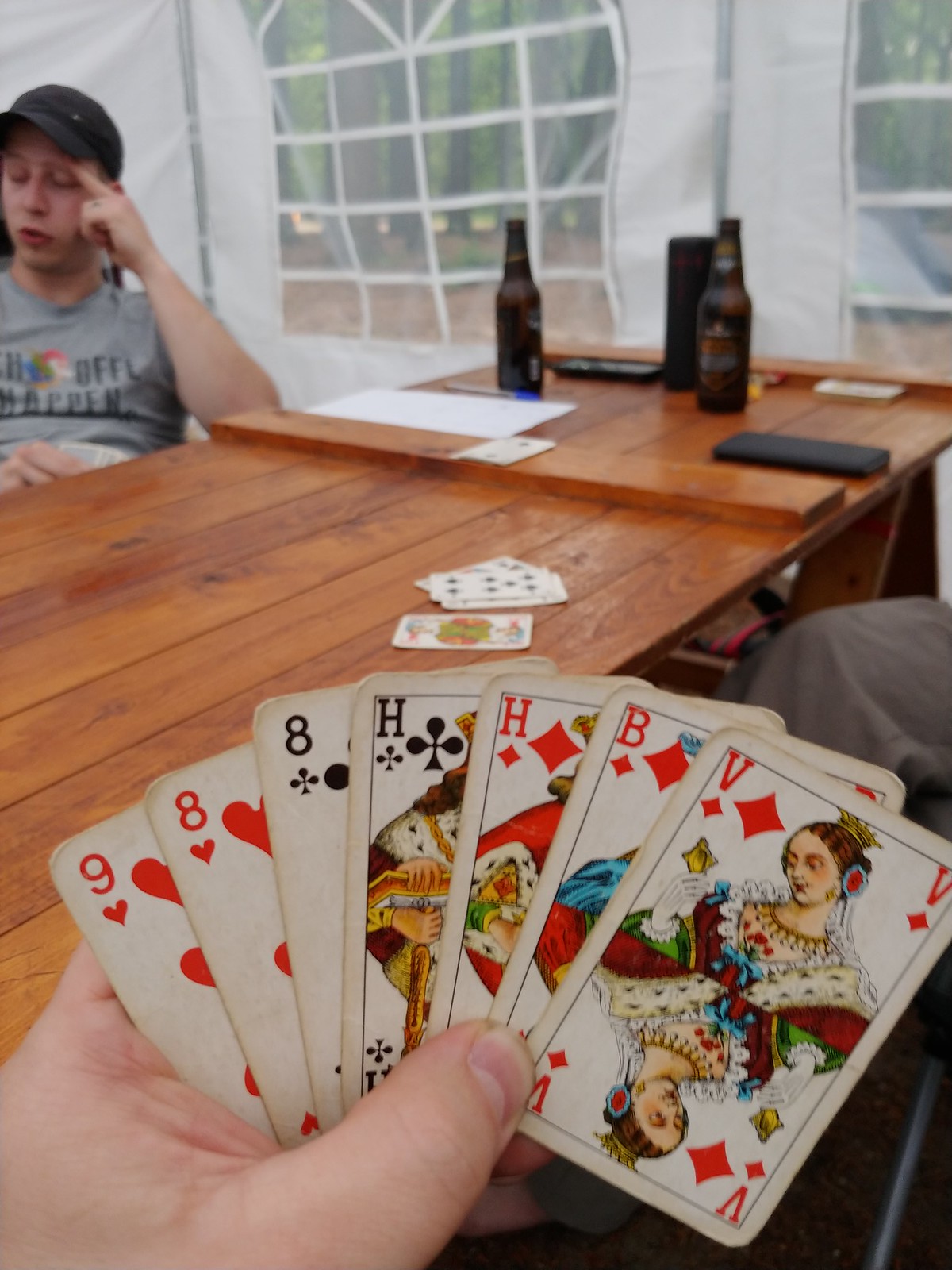In the foreground, a hand holds a fan of cards consisting of the Nine of Hearts, Eight of Hearts, Eight of Clubs, King of Clubs, King of Diamonds, Jack of Diamonds, and Queen of Diamonds. Intriguingly, the King, Queen, and Jack are marked with the letters H, V, and B respectively, rather than the traditional K, Q, and J. The scene is set on a wooden slat table, where four cards rest in the center. At the far end of the table, near a wall, there are a couple of brown beer bottles next to white-framed windows. Across the table from the hand, a young man in a gray t-shirt and black baseball cap sits with his left elbow on the table, his head resting against his pointed index and middle fingers. He glances down and slightly to his right while holding his own hand of cards in his right hand, positioned to his left, not focusing on them.